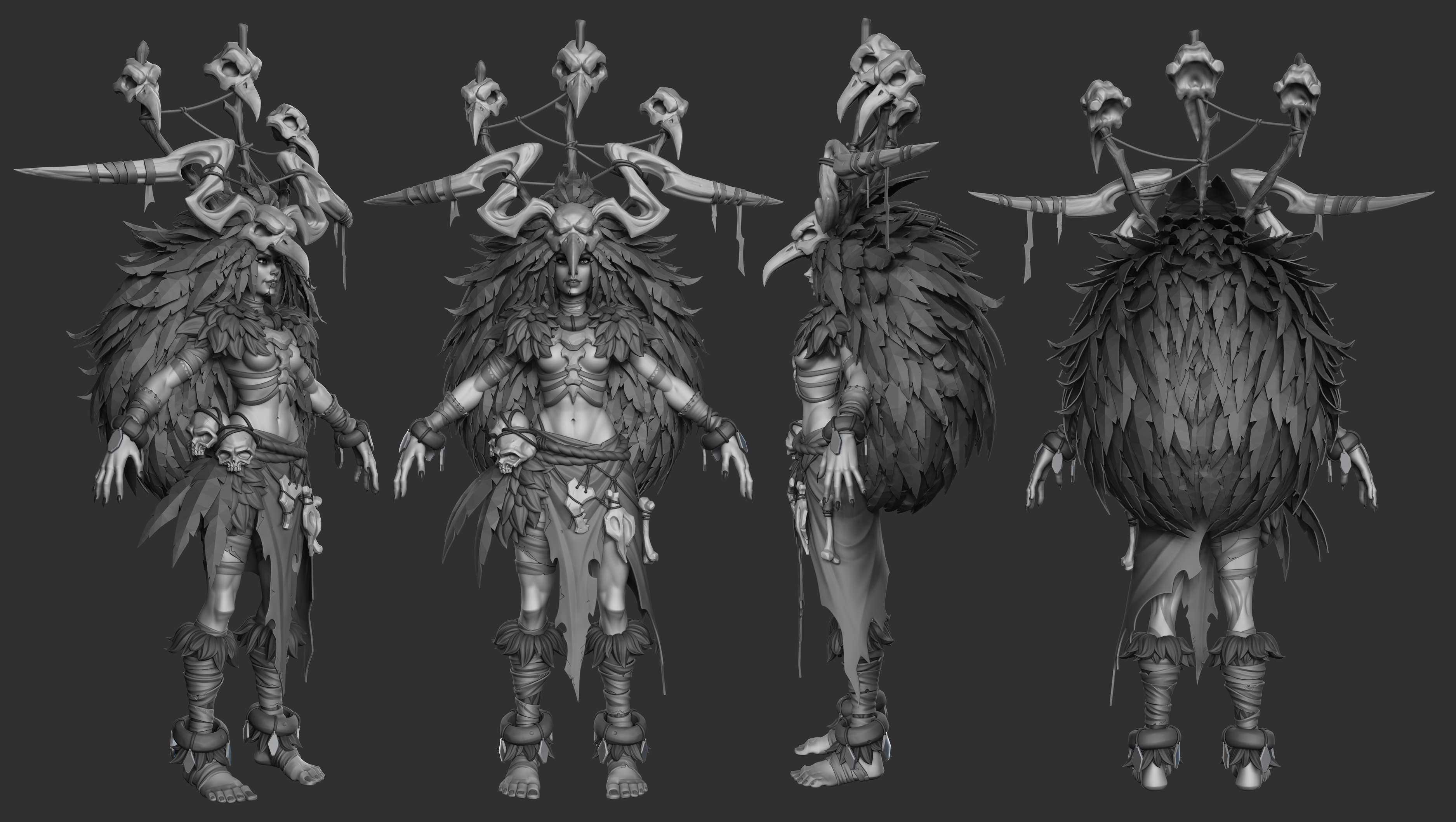The black-and-white image is a highly detailed 3D render of a single female character depicted from four different angles against a solid dark gray background. The character is elaborately dressed in a tribal-inspired costume, highlighted by a striking headpiece adorned with three bird skulls and an antler extending outward, along with numerous feathers. The headpiece features what resembles the face of an eagle perched prominently over her forehead. From left to right, she is shown in varying poses: first, she faces right with her arms extended to the sides; next, she faces the viewer head-on; then, she turns to face left; and finally, her back is to the viewer, revealing a large feathery element reminiscent of a giant backpack. Additional details include decorations on her barefoot and leafy adornments around her legs, contributing to her natural, bird-like appearance.